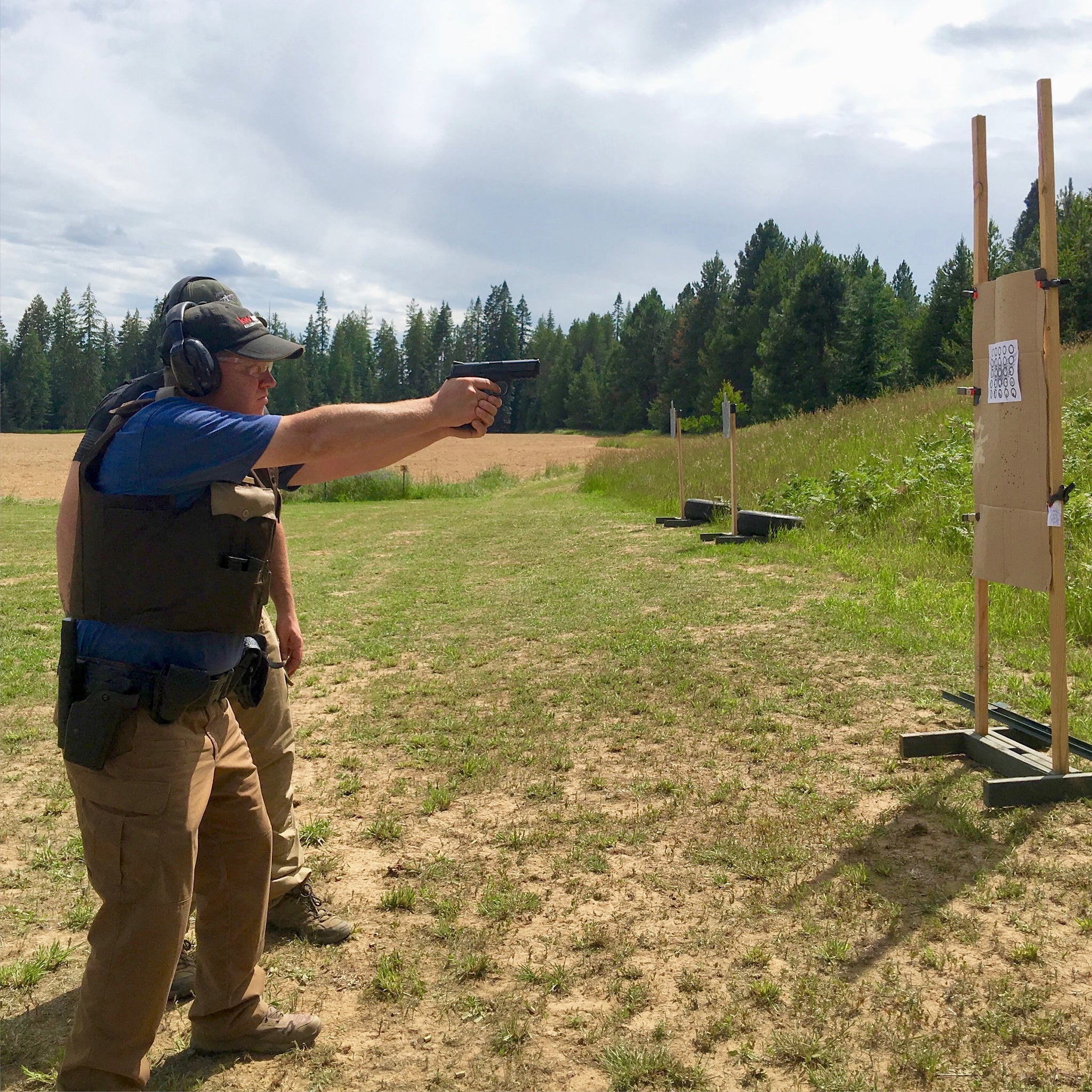In the photograph, two men are at a shooting range with a background of clear blue skies and an expanse of green trees that look like pine. The man in the foreground is the focal point, wearing a blue short-sleeve shirt, a dark green snapback hat with black ear protection muffs, a green bulletproof vest, and a utility belt with holsters. He’s dressed in khaki cargo pants and light brown boots. His arms are extended forward, aiming a small black pistol, likely a nine-millimeter, at a training target about 10 to 12 feet away. The target comprises a piece of paper positioned on cardboard, clamped onto two wooden posts. Behind him, partially obscured, stands another man also wearing a hat and protective ear coverings, a blue shirt, and khaki cargo pants. Distant trees form a green backdrop under a sky scattered with white clouds, with an extended yellow crop field visible in the background. The ground around them appears grassy and bushy, punctuated by a few black tires resting on targets.